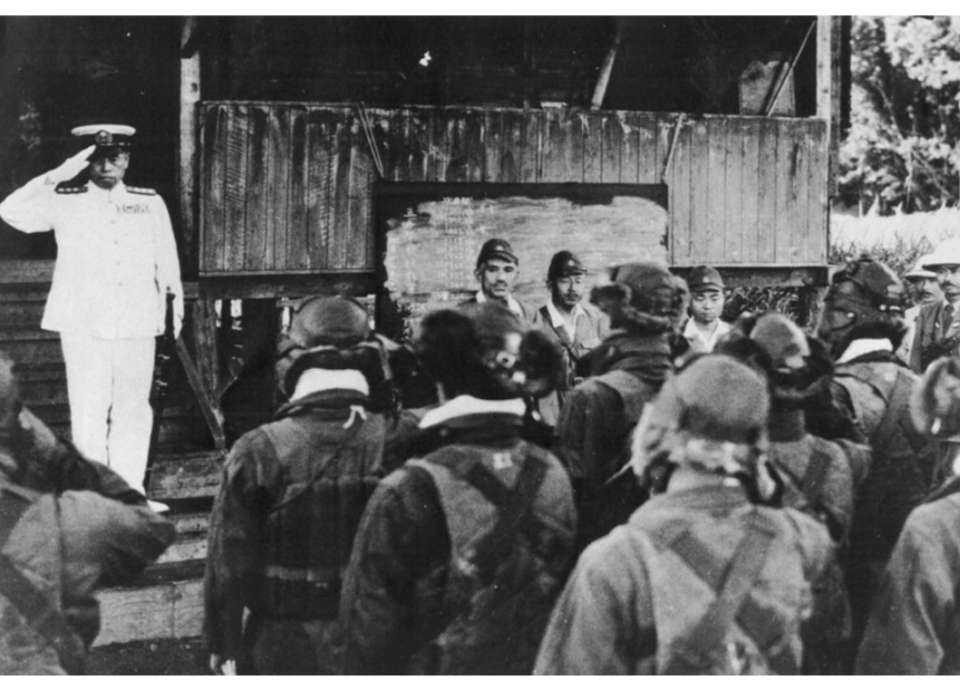This black-and-white photograph, likely from the World War II era, captures a significant assembly of the Japanese Imperial Army. The scene shows soldiers gathered and attentively listening, as seen from behind them, directed towards a makeshift wooden stage. On this stage, there are four distinct figures facing the camera. To the left, a high-ranking naval officer, possibly an admiral dressed in a pristine white uniform and hat, stands at a formal salute. To the right of him, three additional men are present; two appear to be prominent figures—potentially generals or even Emperor Hirohito himself—addressing the troops. These men are dressed differently from the saluting officer, wearing military attire that includes harnesses and vests, reflective of the era's uniform style. The backdrop hints at a jungle environment, enhancing the impression of a wartime setting. The detailed expressions of the speakers and the solemn backs of the listening soldiers contribute to the powerful and historical significance of the image.